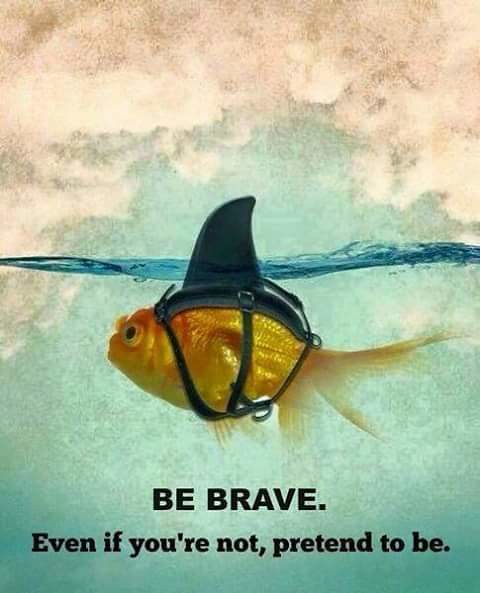The image is a vertically oriented, humorous meme poster featuring a side view of a goldfish swimming to the left. Attached to its body are three harnesses, securing a black, rubber shark fin atop its back, which protrudes above the waterline. The fin gives the illusion of a shark from the surface view. The goldfish possesses a shiny, golden body with its tail extending to the right. The background features a light blue ocean beneath a sky filled with white, fluffy clouds. At the bottom of the poster, bold black text reads "BE BRAVE," followed by "Even if you're not, pretend to be" in slightly smaller font. This playful image encapsulates the notion of courage, even if it means faking it, illustrated by the goldfish's attempt to appear as a fearsome shark.